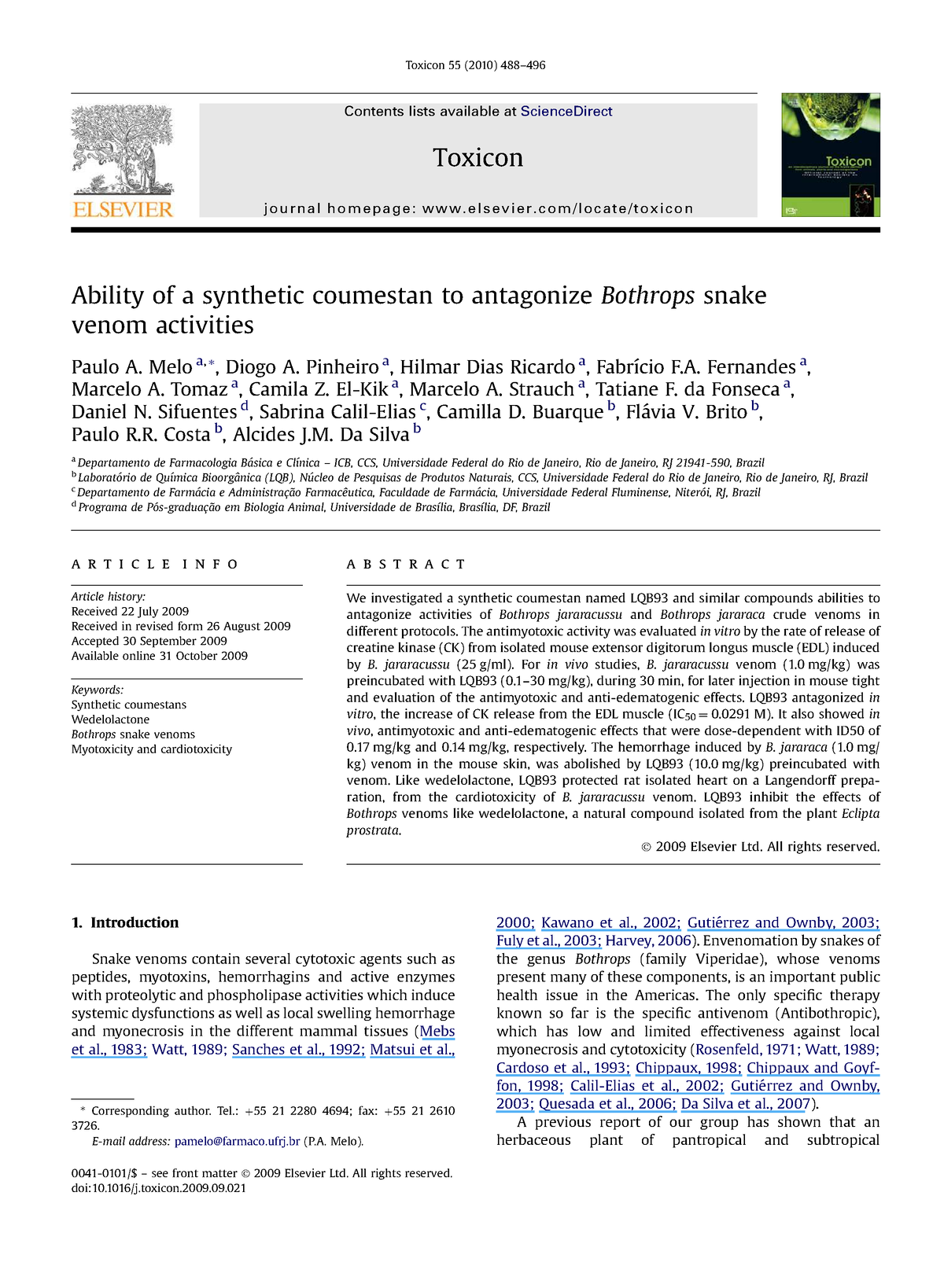This image depicts a screenshot from an academic journal article. The header at the top center reads "Toxicon 55(5), 2010, 488-496" with a single horizontal line beneath it. Below, a gray box contains a hyperlink text, "Contents list available at ScienceDirect," indicating where the full content can be accessed online.

In the middle of the page, the journal name "Toxicon" appears prominently with a note about the journal's homepage URL. On the left side of the page, there's clipart of a tree with "Elsvier" in orange text, and on the right, a thumbnail image depicting a book with green and black colors.

The article's title, "The ability of synthetic coumestrol to antagonize bothrops snake venom activity," is bolded beneath the header, suggesting the research involves synthetic compounds potentially neutralizing snake venom. Authors’ names and affiliated departments are listed, indicating a collaborative research effort involving around 12 individuals. 

On the left side, an "Article Info" section details the article's history, including the dates it was received and accepted, and relevant keywords. 

Below this, the article is structured with an abstract spanning three paragraphs, followed by an introduction and segmented content organized by books and publication years.